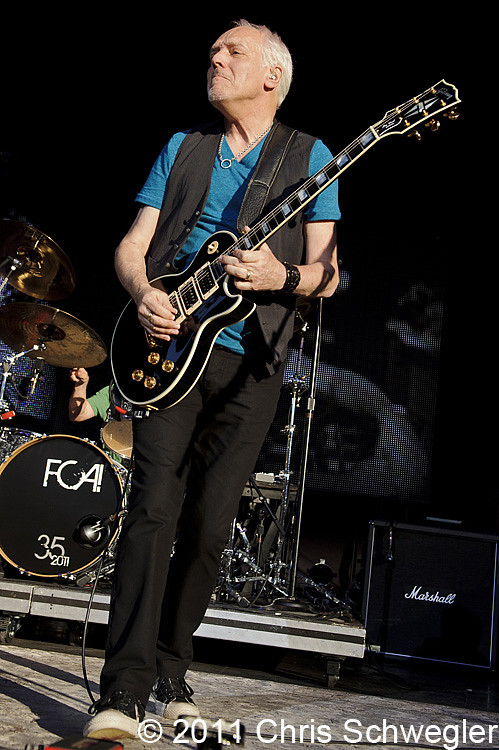In a dynamic outdoor performance, a musician takes center stage, dramatically tilting to his right while strumming a black electric guitar. His attire includes black pants, black sneakers with white soles, an aqua blue V-neck short-sleeved shirt, and a leather-like black vest. With his right foot raised and his head slightly turned upwards as if he’s lost in a powerful guitar riff, his eyes closed, he embodies the essence of rock. Behind him, a drummer is partially visible, seated at a black drum set adorned with cymbals. To the left of the guitarist, a Marshall speaker stands prominently with its logo displayed in white. The stage itself is gray, but the backdrop is a deep black, creating a striking contrast. The lower right-hand corner of the picture bears the photographer's mark, "© 2011 Chris Schwegler," indicating the moment's capture in 2011.